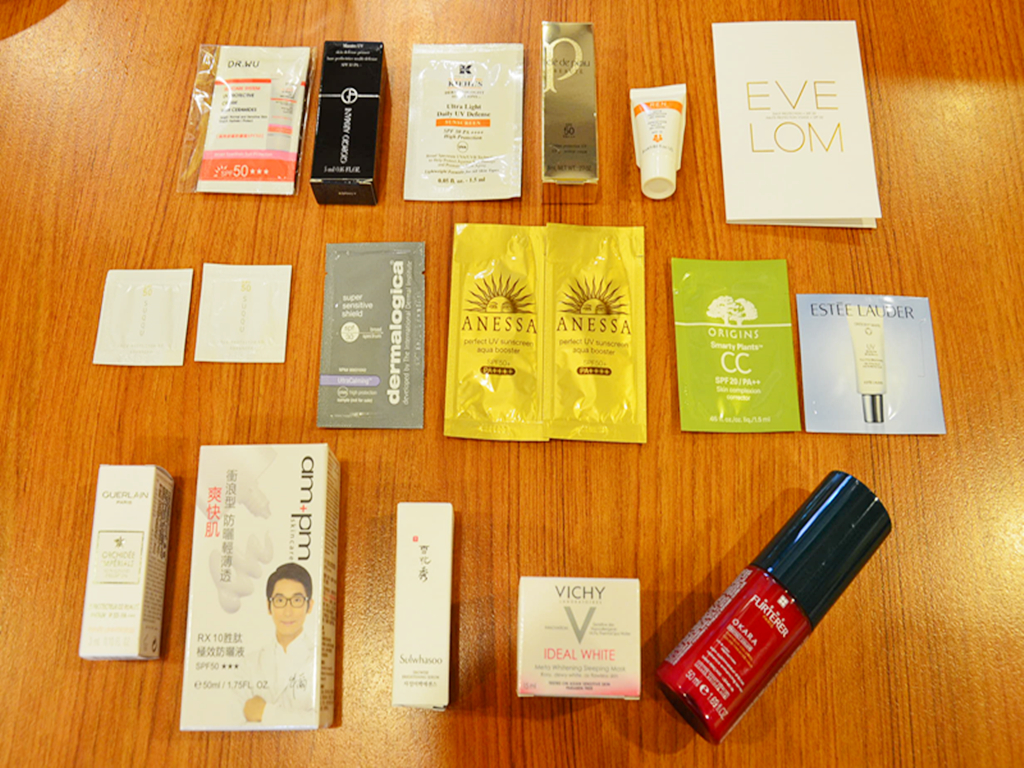On a light medium brown wooden table, a variety of hair and facial products are arranged meticulously. At the top, there's a sunscreen bottle which is flanked by two more containers of what appear to be facial products. Nearby, a sophisticated black box sits alongside a sleek white package and a robust brown box. A luxurious lotion or cream in a white tube is prominently visible, labeled with "Eve Lom." An accompanying card suggests it may contain a perfume sample.

Below this, the next row features two pristine white packages, possibly containing lotion or serum intended for squeezing out. A gray package is placed next to them, followed by two vibrant yellow packages with "Anessa" written on them in bold letters. The sequence continues with a green package adorned with "CC" and "Origin" inscriptions, and an "Estee Lauder" card, inferred to possibly hide another perfume sample.

Among the assortment, a white box branded with "A-M-PM" and several Chinese symbols stands out, leading to another white box also inscribed with Chinese symbols. Completing the organized display, a white box labeled "Vichy Ideal White" is situated next to a strikingly vivid red nail polish bottle. This meticulous arrangement of diverse beauty products creates an enticing and visually appealing presentation on the wooden tabletop.